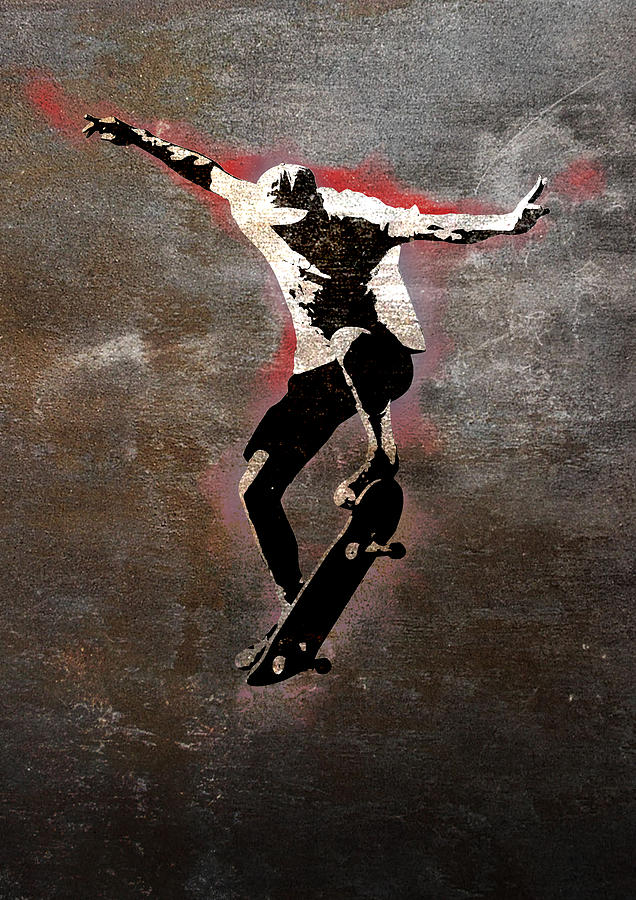This image showcases graffiti art featuring a minimalist, stencil-style depiction of a skateboarder performing an ollie. The background is a patchy, grainy mix of gray, brown, and black, with streaks of white, and a red aura subtly outlining the figure. The skateboarder, rendered in a striking silhouette, wears a white shirt, white hat, black shorts, and tennis shoes. They are captured mid-air, with the skateboard tilted, its front nose up and tail down, wheels clearly visible. The skateboarder's balance is emphasized by their outstretched arms: the left hand with two fingers lifted upwards, and the right hand extended straight outwards. This artistic piece creates the impression of the figure floating, devoid of any ground, highlighting the dynamism and fluidity of the movement against the contrasting, textured backdrop.